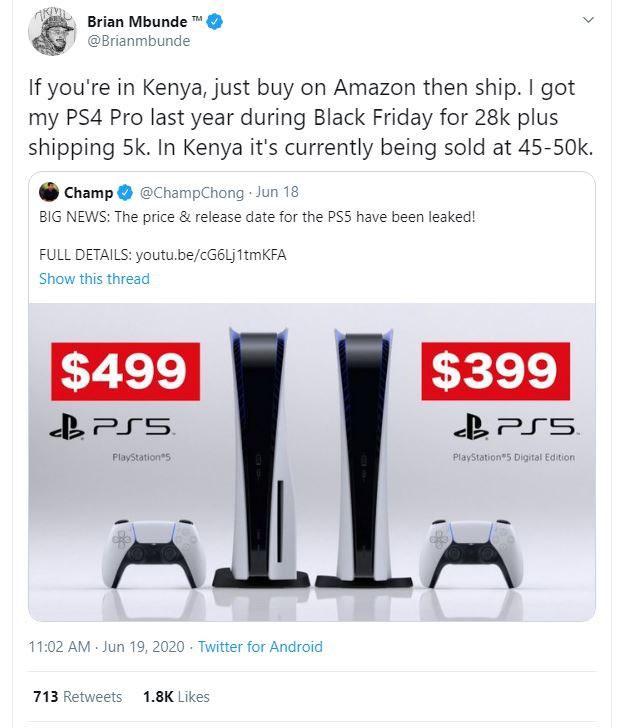This is a detailed screenshot from a smartphone displaying a series of tweets on X, formerly known as Twitter. The user is Brian M. Bunday, identified by his handle @BrianMBunday, which includes the letter "M" and the last name Bunday spelled B-U-N-D-E. His profile photo appears to feature him wearing a ball cap. Brian M. Bunday has a blue verification checkmark.

In Brian's tweet, he shares advice for those in Kenya to purchase items on Amazon and then ship them over. He recounts his experience buying a PS4 Pro for $28K plus $5K in shipping during Black Friday, noting that it is currently priced between $45K to $50K in Kenya.

Following Brian's post, a verified user named Champ, with the handle @ChampChong, replied on June 18. Champ's tweet announces significant news regarding the price and release date for the PS5, accompanied by a YouTube link for further details. The tweet invites readers to view the entire thread for more information.
 
The screenshot includes images depicting the PS5 and its controllers. One image shows the regular PS5 model priced at $499, while another shows the PS5 Digital Edition priced at $399. The timestamp for this activity is 11:02 AM, June 19, 2020, and it was posted via Twitter for Android. Brian Bunday's tweet has garnered 713 retweets and 1,800 likes.